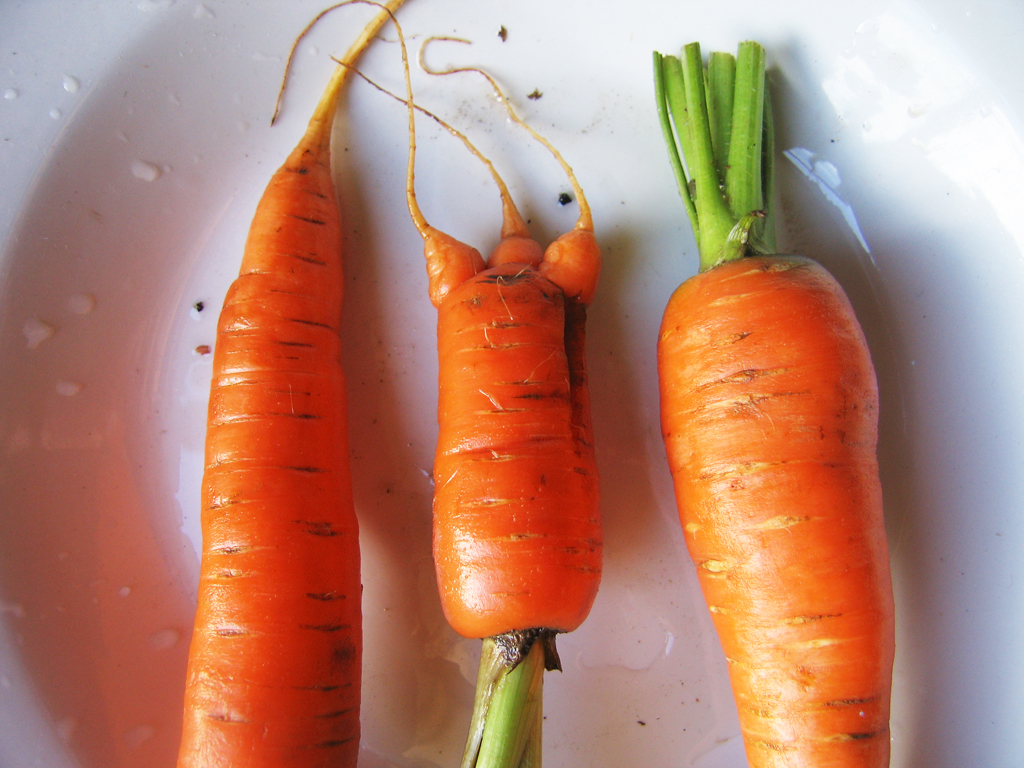This is a close-up photograph of three freshly pulled carrots, arranged horizontally, on a white dish with a slight dip in the middle. The dish is speckled with dirt and droplets of water, indicating the carrots were recently rinsed but not thoroughly cleaned. The carrot on the left is fully orange with only the tapered tip visible. The middle carrot is the shortest, around three inches long, with a green stem at the top and three small, root-like offshoots at the bottom, and still has thin, straggly root hairs. The carrot on the right, the longest, has the green foliage prominently displayed, although the very tip of this carrot is cut off in the picture. All three carrots exhibit natural imperfections, including hash marks and remnants of yellow, adding to their freshly harvested appearance. The image captures the organic essence of the carrots, the texture of the soil, and the glistening water droplets.